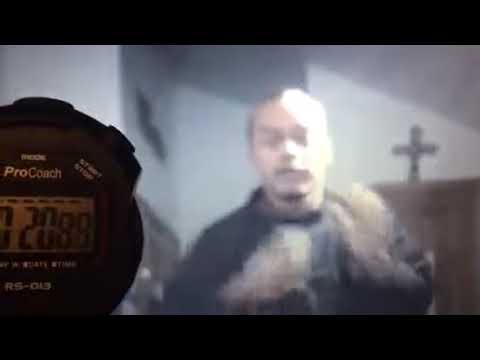This image is a very blurry, dark photograph that appears to capture a scene from a church. In the center, there is a light-skinned man who may be a priest or monk, dressed in a black outfit with his hands raised in front of his chest. Behind him, slightly to the right, is a podium with a cross, set against a white wall that features a visible arch, suggesting a church setting. The background is hazy, making it difficult to discern fine details.

To the left of the priest, there's a sharp contrast with a plastic digital stopwatch, labeled "Pro Coach" in white letters at the top. The stopwatch displays the time as 20.89 seconds. Additional minor details include smaller, hard-to-read lettering and buttons labeled "Start" and "Stop." The entire image is framed with rectangular black borders at the top and bottom, giving it a letterboxed appearance.